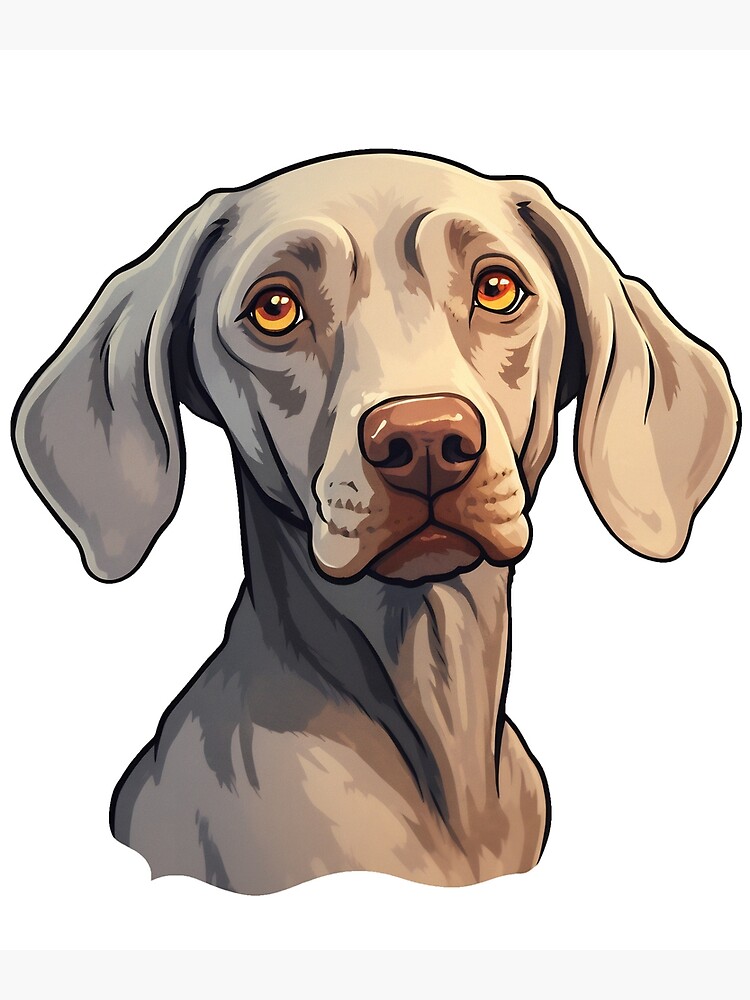This is a colored illustration of a mid-sized dog with a light tan and light brown coat, set against a plain white background. The depiction includes only the upper part of the dog's torso, primarily focusing on the neck and head. The dog appears to be looking straight forward with a sad and welcoming expression. Its golden-brown eyes, which have yellow irises, convey a sense of melancholy. The dog's ears are large, floppy, and folded over, adding to its expressive demeanor. The nose is a dark brown, while the snout and surrounding fur have varying hues of brown. There is shadowing on the left side of the dog's neck, indicating that the light source is coming from the upper right of the image. While there is some detail in the texture of the fur, the overall color palette is simplified, focusing on different shades of brown. The breed of the dog is not clearly identifiable, though it resembles a beagle, a Labrador, or possibly a golden retriever.